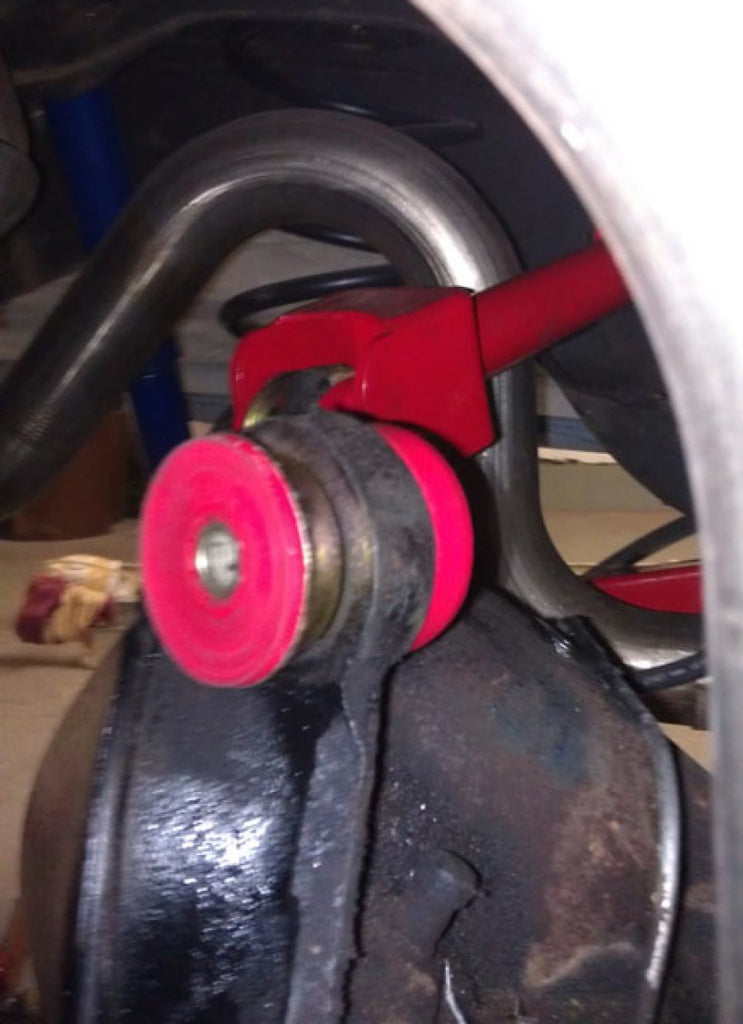The image depicts a detailed close-up of a specific part of a car’s mechanical system, captured indoors. At the top of the image, a silver tube forms an upside-down U-shape, resembling a backwards S. Directly beneath this structure is a red arm extending from the right, gripping a silver gear. This gear is encircled by a black rubber belt and features hot pink end caps. Below the gear, there is a piece of black, oily metal. The background shows a tan floor, with a black seat visible behind the main components. There is also a brown cardboard box, and a nearby object with gold, white, and blue details. The whole scene suggests the wheel has been removed, exposing the metal parts, some of which are rusty.